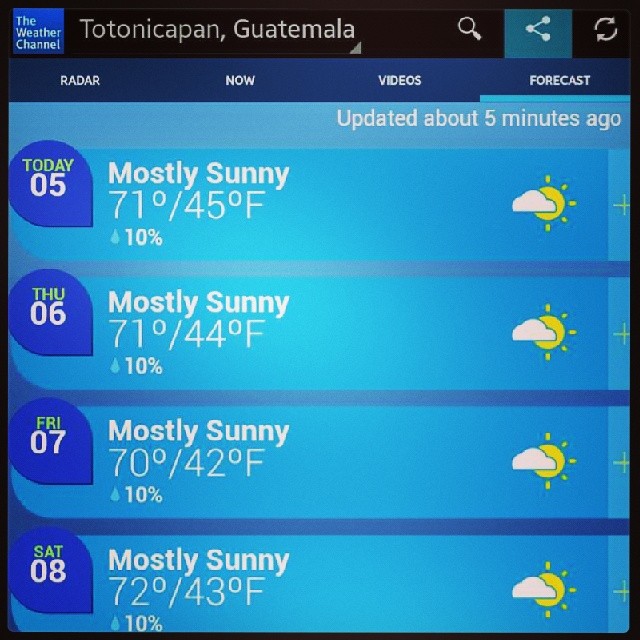The screenshot depicts a weather app providing detailed weather information for Totonicapán, Guatemala. At the top right, there's "The Weather Channel" logo in a black square with a green square behind it. Next to it is the location name in a black banner. Adjacent to the banner, there are icons for an hourglass, a share symbol, and a reload symbol. Below this, a blue navigation bar showcases options such as "Radar," "Now," "Videos," and "Forecast" in white text.

The main section is divided into four rows, each representing a different day:
1. **Today (05)**: Mostly sunny with a high of 71 degrees and a low of 45 degrees. There is a 10% chance of rain, indicated by a raindrop symbol.
2. **Thursday (06)**: Mostly sunny with temperatures ranging from a high of 71 degrees to a low of 44 degrees, and a 10% chance of rain.
3. **Friday (07)**: Mostly sunny with a high of 70 degrees and a low of 42 degrees, and a 10% chance of rain.
4. **Saturday (08)**: Mostly sunny with a high of 72 degrees and a low of 43 degrees, and a 10% chance of rain.

Each day is represented with an icon showing a white cloud partially covering a yellow sun. To the right of the weather details, there are green plus signs.